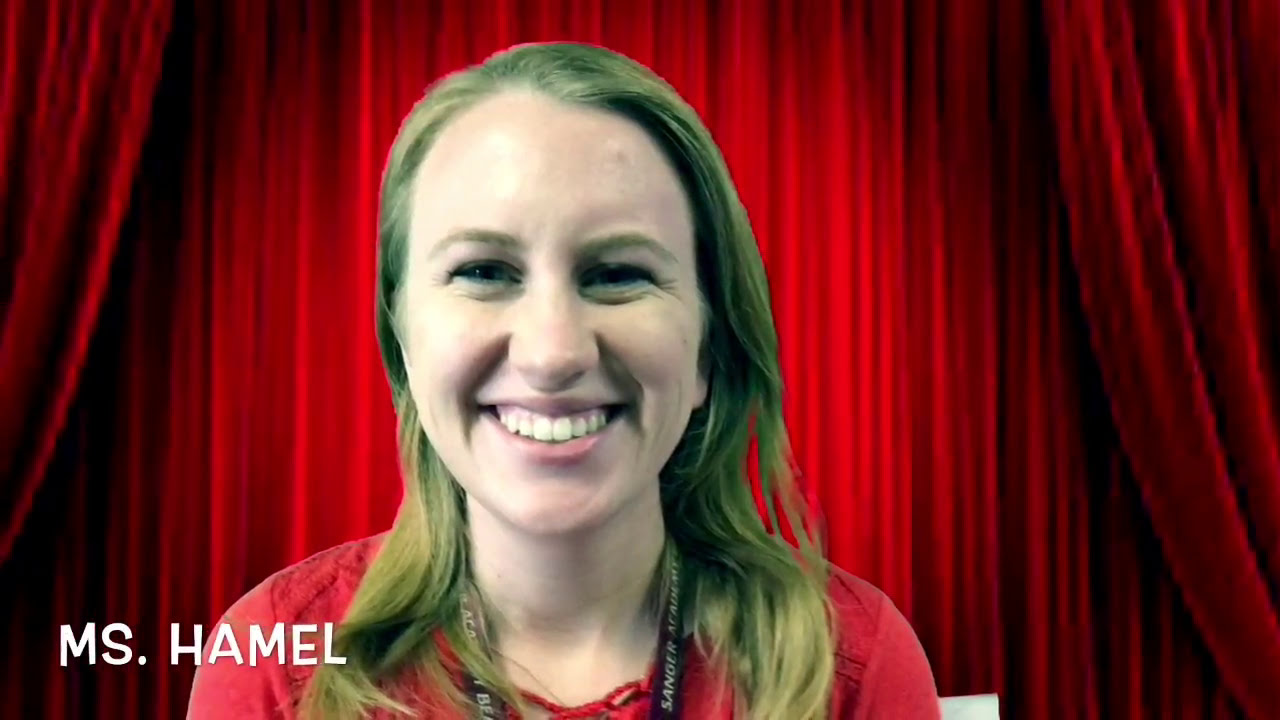In this digitally enhanced, horizontally rectangular image, we see a Caucasian woman with thin blonde eyebrows and long, wavy blonde hair draped over her shoulders. She wears a light red or pinkish t-shirt and a lanyard around her neck, which displays the words "Sanger Academy." The woman, potentially a teacher named Ms. Hamill, as indicated by the white text in the lower left-hand corner, is smiling broadly, showing her white teeth.

She appears to be sitting in front of a backdrop designed to look like the red curtains of a theater. The deep red curtains, complete with drapes on the left and right, provide a dramatic setting. A spotlight shines down the center of the curtain, enhancing the theatrical ambiance. This setup, likely part of a virtual meeting platform such as Zoom, suggests that Ms. Hamill might be addressing her class or audience remotely.